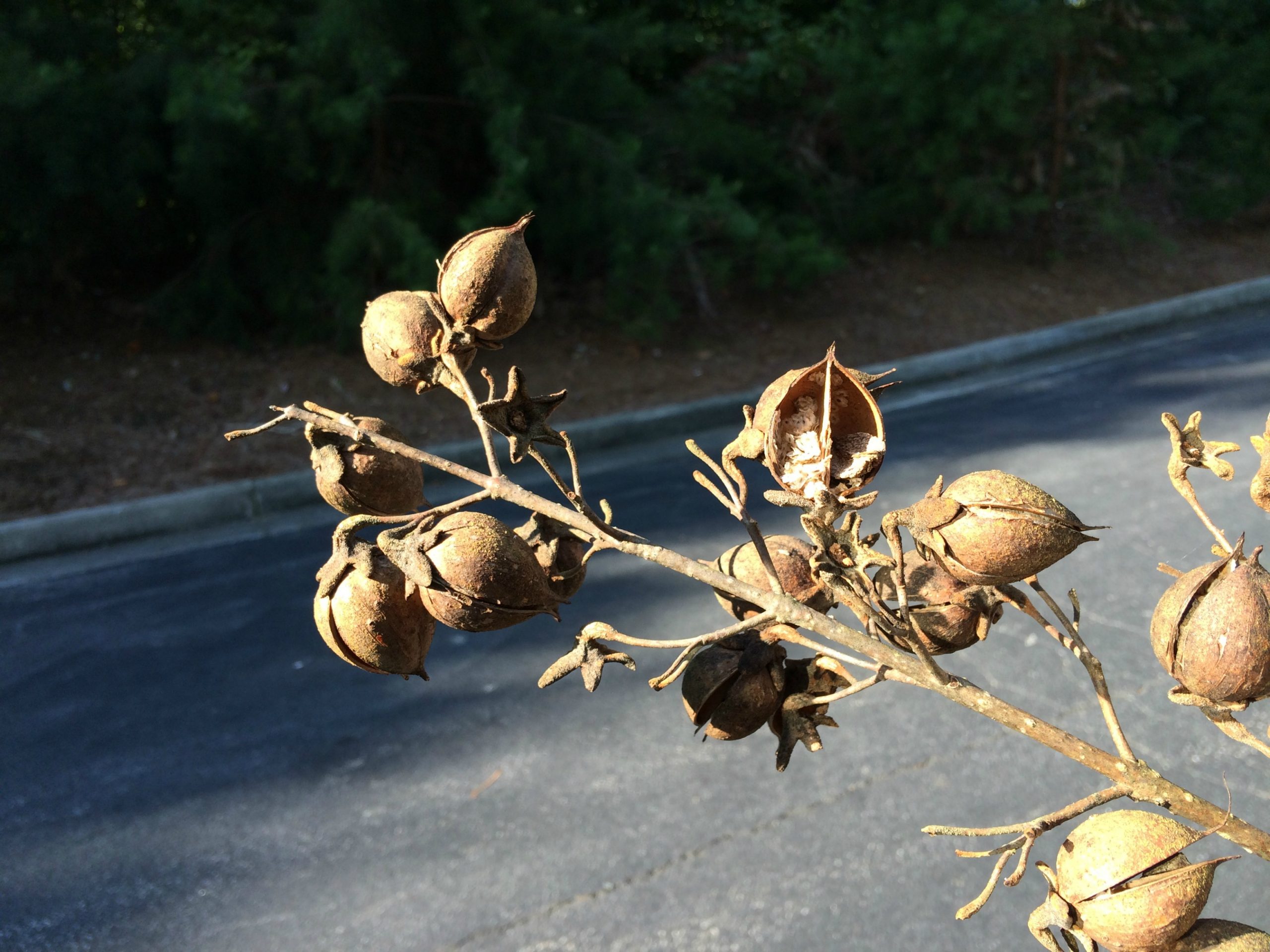The photograph features a prominent dried branch with at least 11 seed pods, some opened to reveal two or three internal chambers, while others remain intact or have already fallen. These seed pods, resembling rosebuds or alien mouths slightly ajar, dominate the foreground. The branch hangs above a gray roadway, accompanied by a visible sidewalk and curb. Beyond the curb, there is a strip of soil leading into a darkened area filled with trees and shrubs. The background appears barren and nearly moon-like in its desolation, with an upper left section of the image fading into complete darkness. No people or vehicles are present, emphasizing the eerie and almost lifeless appearance of the scene.